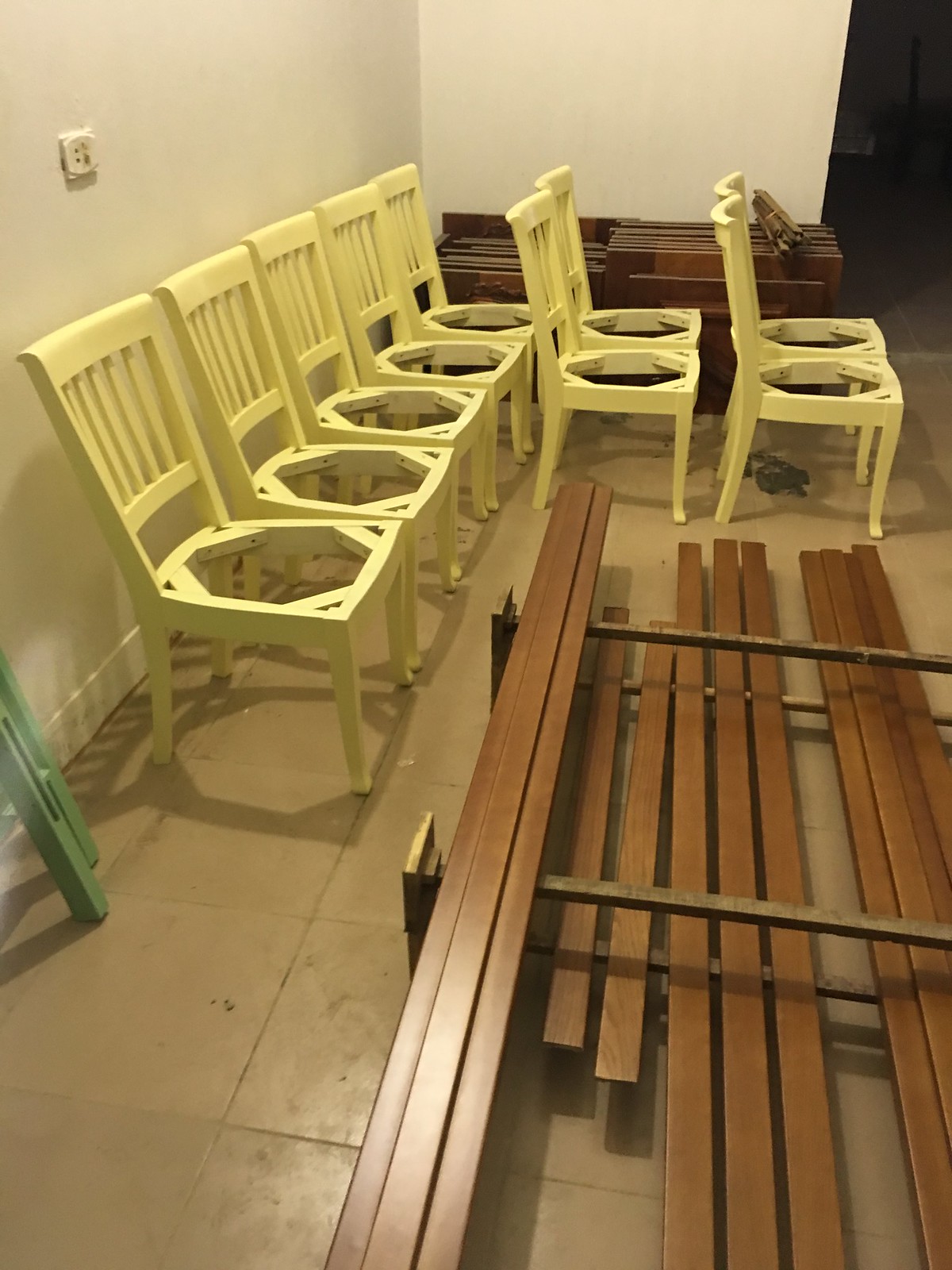The photograph depicts a white room with a beige-tiled floor, showcasing an arrangement of pale pastel yellow wooden chairs, each missing its cushion and thereby exposing a hexagon or octagon-shaped hole in the center of the seat area. The chairs are lined up side by side against the wall, with straight-slatted backs. There are five chairs positioned at the back, two in the middle, and two more towards the front, all leaning against the wall. In front of these chairs are several planks of dark brown stained wood, some of which are leaning against the wall, while additional black slats or rods are scattered on the floor towards the middle and lower right side of the image. The scene suggests an assembly area potentially related to furniture crafting.